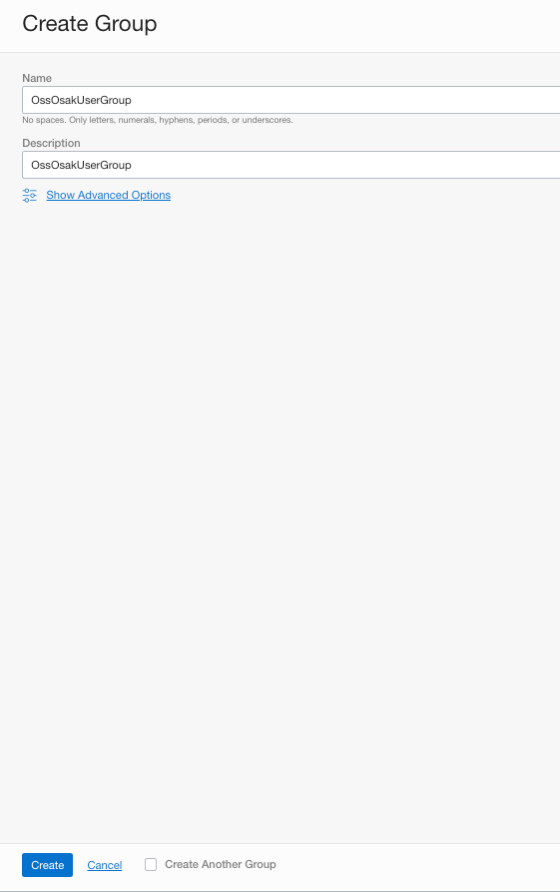The image displays a webpage form for creating a group. The top of the form prominently features the title "CREATE GROUP" in capitalized letters. Below the title is a single-line text box labeled "Name," where users can input the name of the group. This field accepts only letters, numerals, hyphens, periods, or underscores, as indicated by the instructions underneath.

Another text box labeled "Description" follows, allowing users to type a brief description of the group. Both the "Name" and "Description" fields are mandatory for group creation.

Below the description box, there is a hyperlink in blue labeled "Show advanced options." Clicking this link likely reveals additional fields for a more detailed group setup beyond the basic name and description.

At the very bottom of the form, there's a blue "Create" button to finalize the group creation process. To the right of this button, there is another hyperlink labeled "Cancel" that allows users to exit the form without saving. There is also a checkbox labeled "Create another group," which, if selected, enables users to immediately start creating another group upon submission.

In summary, this form is designed to facilitate the creation of user groups with fields for the group name and description, and an option for advanced settings to provide further details.